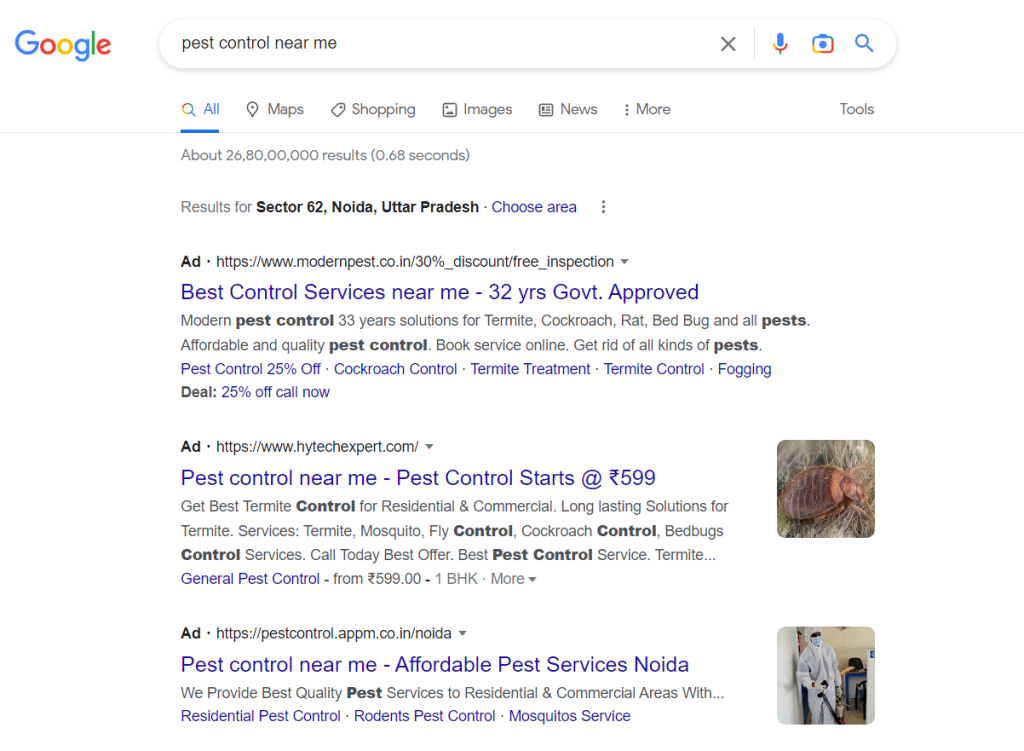This is a detailed caption for an image of a Google search results page:

The image captures a screenshot of a Google search results page. At the top left corner, the distinctive Google brand logo is prominently displayed. Adjacent to the logo, a search bar contains the query "pest control near me." To the far right of the search bar, there is an 'X' icon, followed by a microphone icon, a phone icon, and a magnifying glass icon. The search has returned approximately 268 million results in a swift 0.68 seconds. Directly beneath this information, the page specifies that the results are relevant to Sector 62, Noida, Uttar Pradesh.

The initial three search results are marked with an "Ad" label, indicating they are advertisements. The first link, labeled "Government Approved Pest Control Services Near Me - 20 Years Experience," directs to the website modernpest.co.in. The second link, titled "Pest Control Near Me," points to mytechexpert.com. The third link, "Affordable Pest Services in Noida," directs users to pestcontrol.appm.co.in. Notably, the second and third links include thumbnail images positioned to the right of the text, presumably offering a visual glimpse into the services provided.